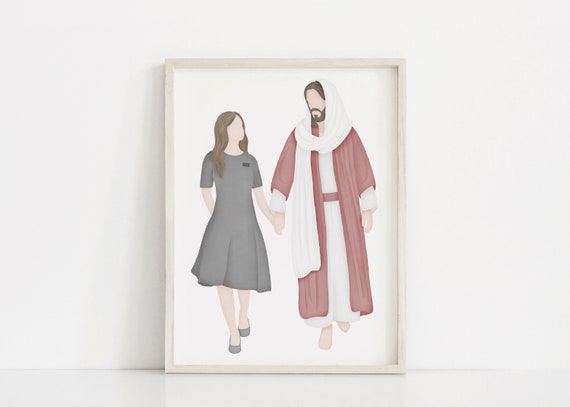The image features an illustration set within a light wooden frame, positioned against a white background which could either be a wall and a table or a floor. At the center of this illustration, with its own white backdrop, is a depiction of a figure that closely resembles the traditional portrayal of Jesus and a woman. The Jesus-like figure stands to the right, adorned in a white robe layered with a red cloak, a brown belt, and a white scarf used as a headpiece, revealing his light skin, brown hair, and brown beard. He walks barefoot, his expressionless face tilted slightly towards the woman beside him, emphasizing their connection. Jesus is shown holding the woman's left hand with his right.

The woman, who also has light skin, has long brown hair cascading past her shoulders and wears a blue dress with matching shoes. Lacking facial features, she walks in tandem with the Jesus figure, her left hand reaching out to hold his. Her right hand is subtly tucked behind her back, reinforcing the impression of movement towards the viewer. This serene and sacred tableau, free of text, suggests a symbolic or religious theme, potentially representing the supportive presence of Jesus in one's life journey.